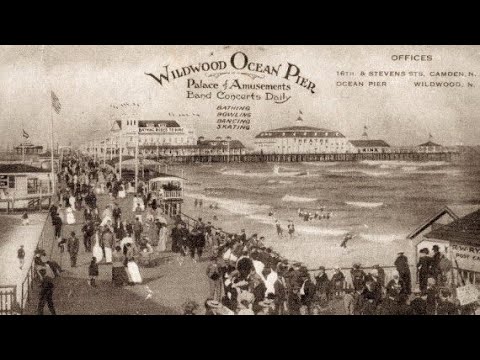This vintage black-and-white illustration depicts the bustling Wildwood Ocean Pier, prominently labeled "Palace of Amusements" at the top. On the right side, it notes the location of offices, along with the address. The scene portrays a lively pier filled with around 100 people in various attire walking up and down, framed by two large buildings with American flags on the left. Several other structures overlook the pier, providing a sense of depth and activity. Below the pier stretches a vibrant beach where additional individuals enjoy the waves. Details indicate that the pier was a center for activities such as bathing, rowing, bowling, dancing, and skating, suggesting a fair-like atmosphere. The ocean, depicted in shades of gray, appears somewhat rough, adding to the dynamic feel of the scene. This likely early 20th-century image captures a snapshot of daily life at a popular seaside attraction.